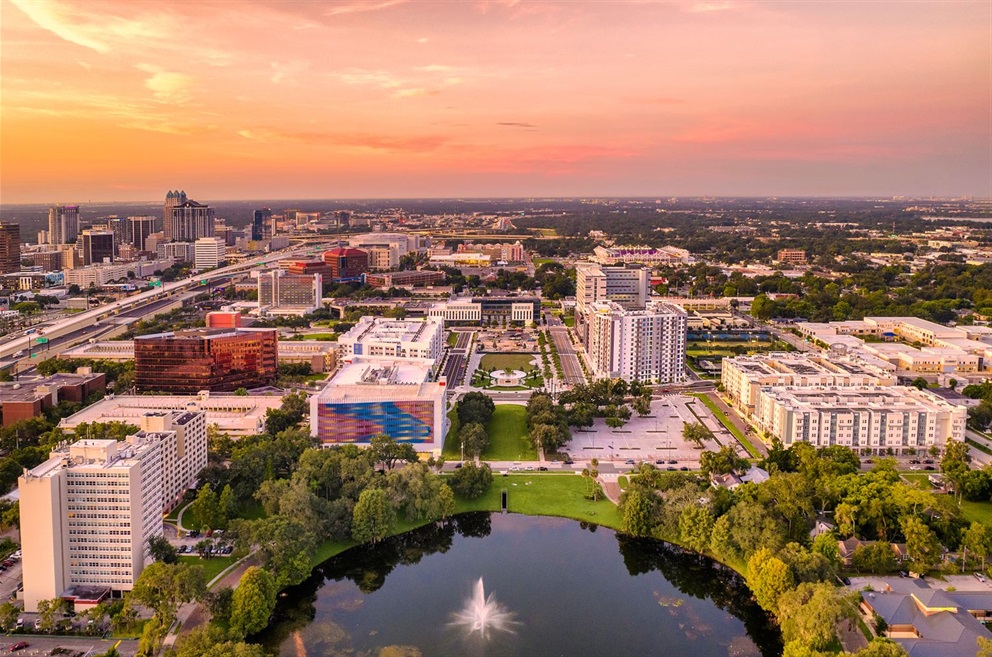The image is an aerial view of an urban area during sunset, bathed in the warm hues of orange, pink, and purple with light cloud cover. In the foreground, a large retention pond with a fountain shooting water up and turning it white is surrounded by a ring of trees and greenery. To the immediate left of the pond, a series of tall buildings—likely apartments or office buildings—are visible, some adorned with colorful murals in shades of red, blue, and gold. These buildings are encircled by a large parking lot. On the right side of the pond, a smaller residential complex, which could be mistaken for a single large house, is nestled among more trees and grass. 

Further out, a main highway with green signs stretches across the left side of the image, separating the pictured area from the downtown core located in the upper left portion, where skyscrapers in varying heights and colors rise against the horizon. Beyond this, the land is flat and expansive. On the far right of the image, the urban sprawl transitions into a more open woodland area. This dense urban scene showcases straight roads and ample green spaces blended efficiently with residential and commercial structures, reflecting the colors of the setting sun in a tranquil cityscape.